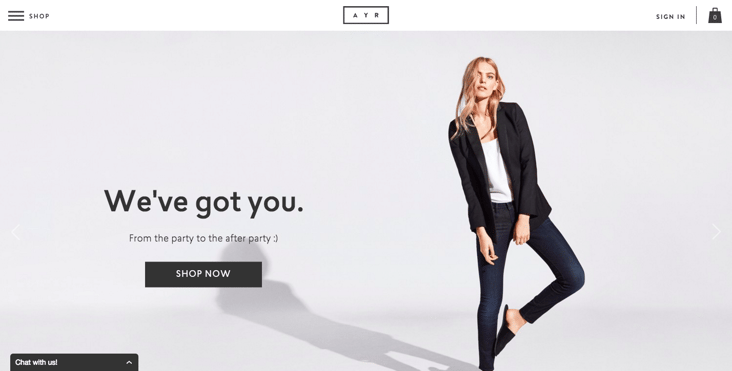The image is a screenshot of a website with a clean, white background. At the very top of the page, there is a menu icon represented by three short horizontal lines, and beside it, the word "SHOP" is prominently displayed in bold, black, uppercase letters. Centrally aligned at the top, a small, thinly bordered black rectangle contains the letters "AYR," also in uppercase and evenly spaced, giving a refined and minimalist appearance. 

On the top right corner, there are the words "SIGN IN" in black, uppercase letters, accompanied by a small shopping bag icon.

The main focus of the image is a woman striking a poised stance; she stands on one leg with her other foot resting against her calf. She is dressed in dark blue jeans and a white top, layered under a sleek black blazer. Her blonde hair partially obscures one of her eyes, adding a touch of casual elegance to her look. She is wearing black slippers and cast a subtle shadow behind her, adding depth to the presentation.

Adjacent to the woman, in large, bold, black letters, the text reads, "WE'VE GOT YOU." Beneath this, in smaller, lighter gray text, it reads, "FROM THE PARTY TO THE AFTER PARTY," accompanied by a small, playful smiley face.

Toward the bottom of the image, there is a gray rectangular button with the text "SHOP NOW" in white, inviting users to take action.